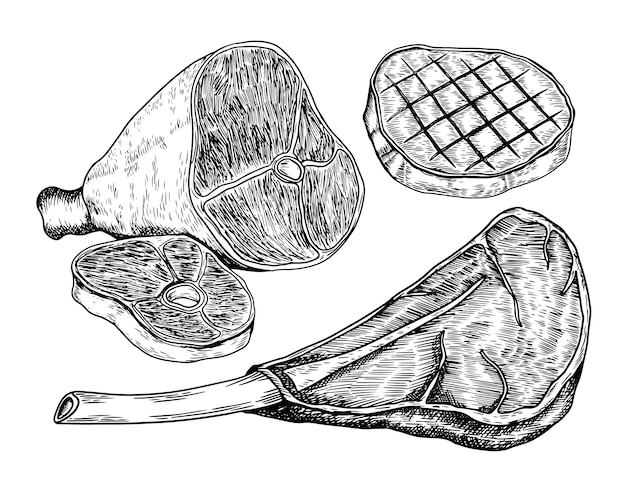This detailed black-and-white ink drawing vividly showcases an assortment of various meat cuts meticulously rendered on a stark white background, devoid of any borders. Dominating the foreground is an impressive tomahawk steak, flaunting its distinctive long bone jutting out, bare and unadorned, contrasted by the succulent meat at the end. To the upper left, a full leg of ham is prominently featured, with a large ham steak sliced from it and laid in front, revealing its cross-section. Just below this, another cut, possibly part of the leg, is visible. The upper right corner is occupied by a circular, boneless pork loin or chop, distinguishable by the intricate cross-hatch pattern etched onto its surface, as if tenderized or seared on a grill. Each cut is intricately detailed, conveying the textures and forms of the meat, appearing almost ready to leap off the page, showcasing the artist’s skill in this hand-drawn, pen-and-ink illustration.